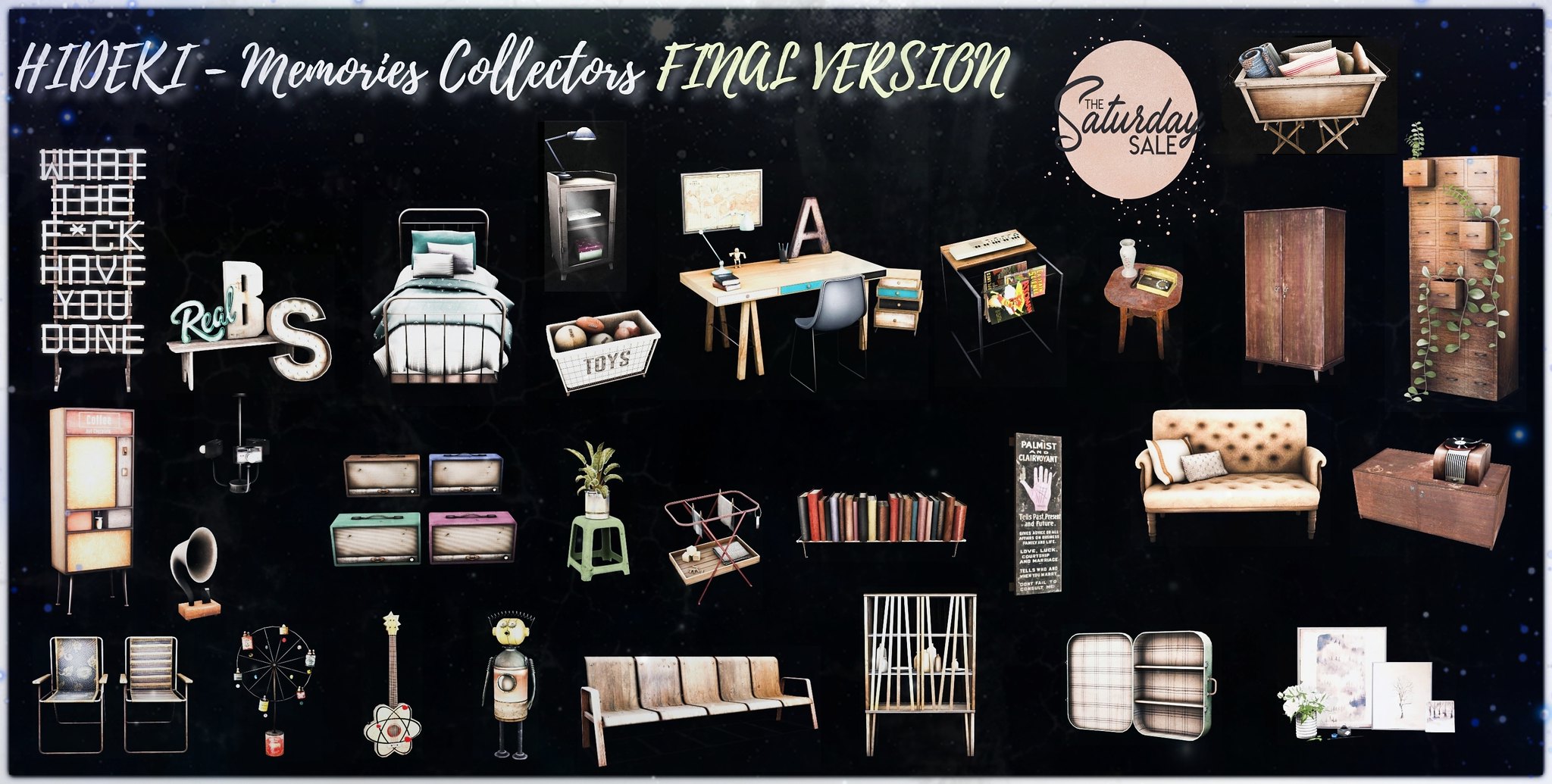This long rectangular advertisement features a collage of various objects against a flat black background, promoting a furniture store called "Hindeki Memories Collections." The top left of the image prominently displays the text "Hindeki.memoriescollections," followed by "Final Version" in yellow, with "Saturday Sale" encased in a circle next to it. Scattered throughout the image are colorful miniature depictions of items such as bookshelves, a chair, a coffee table, a bed, and knickknacks like little guitars and dolls. There's also an array of more specific items, including an easy chair, a toy box, a side table with a lamp, a desk with a monitor, an end table, a cupboard, and a dresser with drawers partially opened to reveal plants. Additional objects such as a horn on a stand, plastic storage holders, a shelf of books, a poster with unreadable text, a sofa with cushions, a coffee table, an open suitcase, and flower arrangements can be observed. Interspersed text elements include phrases like "What the F*CK have you done" on the left side and "real BS" situated nearby. The meticulously detailed array of eclectic items artfully sprawls across this dark backdrop, inviting viewers to explore the myriad of collectible memories on offer at the sale.